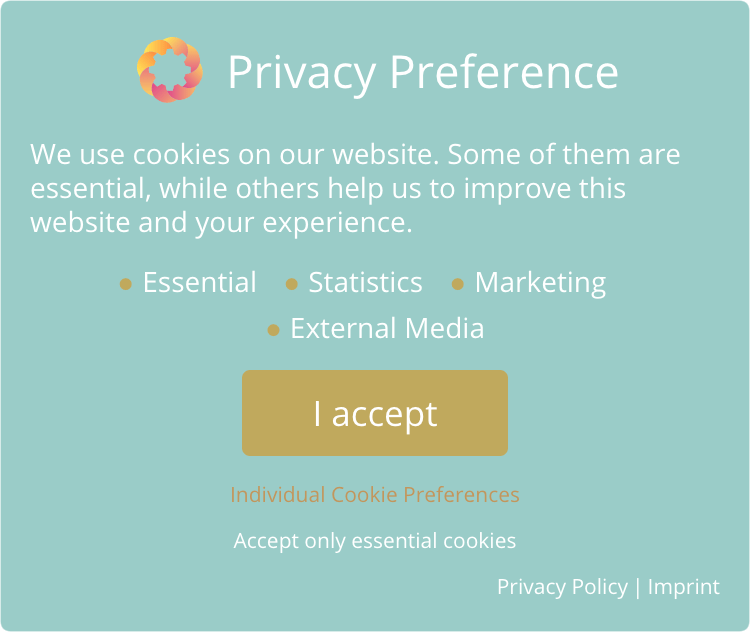This image captures a section of a webpage predominantly featuring a greenish-blue background. At the top, there is a distinctive icon resembling a flower, rendered in shades of orange, yellow, and pink. The heading "Privacy Preference" is prominently displayed in white, larger font.

Beneath the heading, a privacy notice written in white text states: "We use cookies on our website. Some of them are essential while others help us to improve this website and your experience."

Following this text are four bullet points, each marked by a brownish bullet. The bullet points read:
1. Essential
2. Statistics
3. Marketing
4. External Media

Below these bullet points, there is a brownish-colored button with white text that says "Accept." Additionally, another button in the same brownish hue with white text reads "Individual Cookie Preferences." Further down, the option "Accept Only Essential Cookies" is presented in white text.

At the bottom right-hand corner of the image, "Privacy Policy / Imprint" is displayed in white, completing the privacy preferences section.